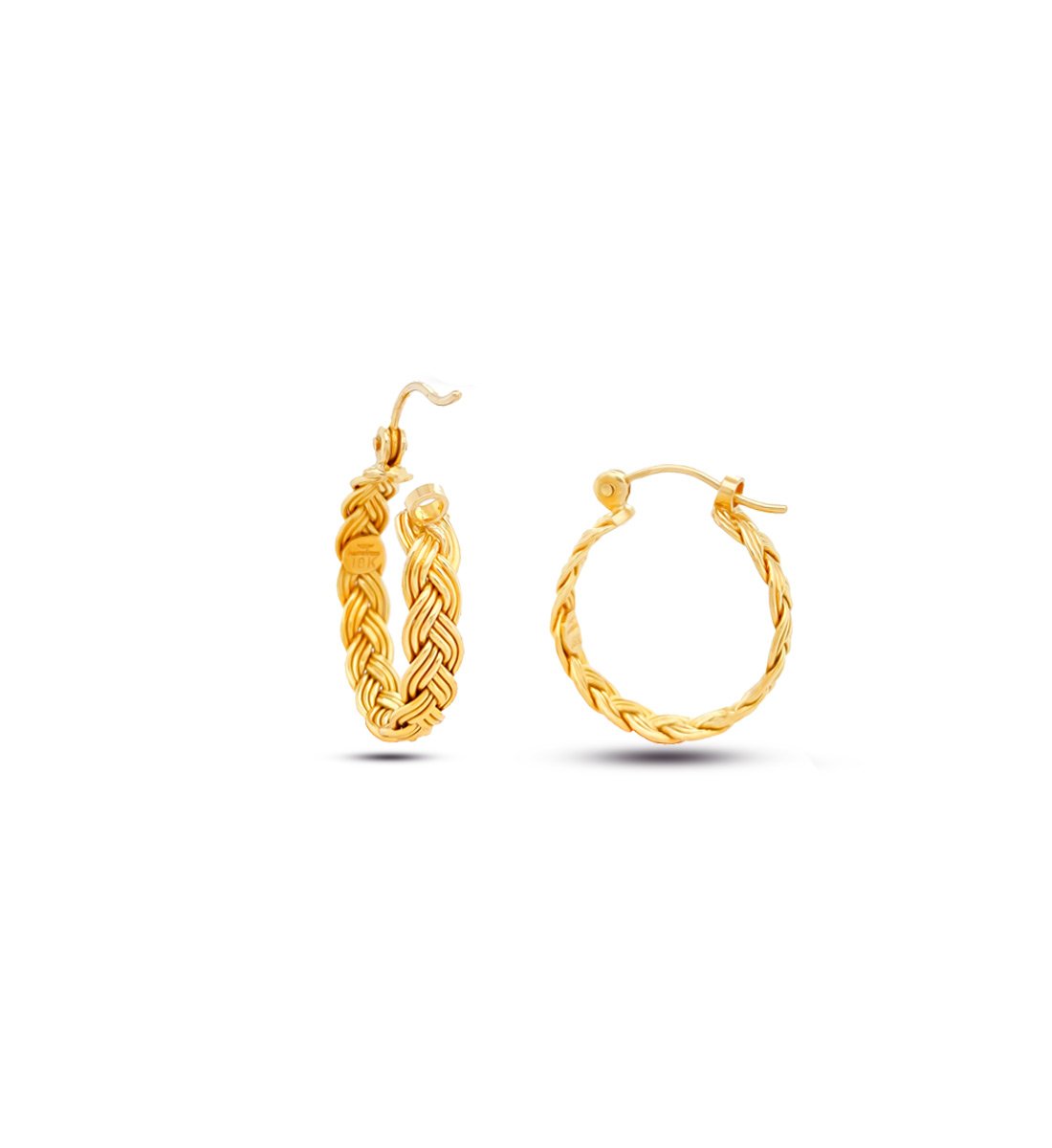This image showcases a pair of gold hoop earrings with a delicate, intertwined rope-like design. Positioned against a stark white background, the earrings create a sharp contrast and are accentuated by digitally-rendered, oval-shaped shadows beneath them, giving the illusion they are hovering. Both earrings feature intricate braiding, resembling three interwoven wires on each side, forming a seamless circular hoop. The earring on the right is shown closed, presenting a nearly perfect circle, while the earring on the left is slightly open, allowing a clear view of the clasp mechanism. The clasps are thin, gold rods designed to secure the earrings through pierced ears. Notably, there is an unreadable marking inside the earrings, suggesting some form of craftsmanship or branding. This meticulous depiction, likely intended for a jewelry advertisement, emphasizes the elegance and precise detailing of the rope pattern, making the earrings the focal point of the scene.